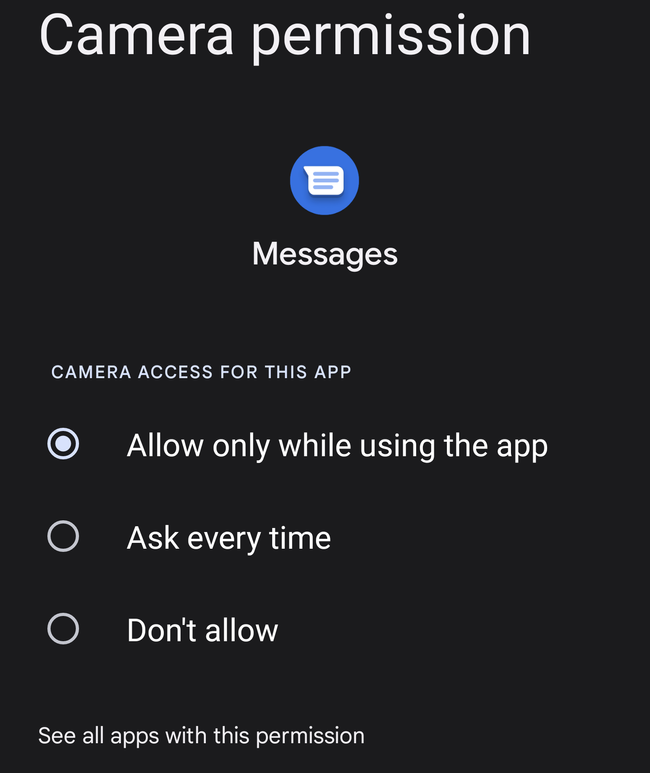A detailed screenshot of a phone's camera permission settings is displayed against a jet-black background. At the top, bold and prominent white letters spell out "Camera Permission," immediately capturing attention. Below this heading, there are several options:

1. An icon featuring a blue circle with a small box and an arrow, symbolizing messages, accompanies these settings.
2. A section labeled "Camera access for this app" is underlined, indicating the active selection.
3. The "Allow only while using the app" option is highlighted and checked, ensuring camera access is granted exclusively during app usage.
4. Two additional options, "Ask every time" and "Don't allow," remain unchecked.
5. At the bottom of the screen, a link labeled "See all apps with this permission" is displayed, offering further permission insights.

The backdrop of the settings menu is uniformly black, while all text, especially the "Camera Permission" heading, is rendered in striking white for high contrast. This combination ensures the menu is both visually appealing and easy to read.